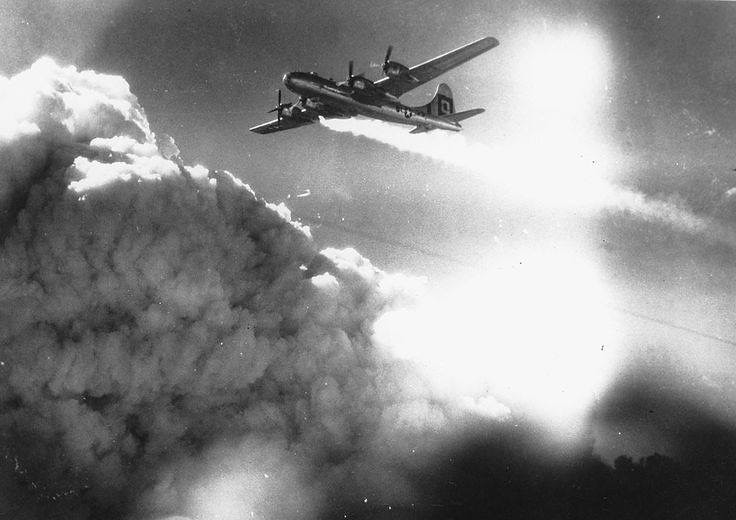In this black-and-white photograph, a wartime setting is depicted with a prominent visual of a military aircraft centered towards the top of the image. The aircraft, a single fighter jet with four propellers at the front, is flying from right to left. There is a noticeable stream of smoke trailing from the right side of the plane, which may be indicative of an engine fire. The background features the sky, dotted with various clouds, some of which form a large, billowing area of smoke that spans across the bottom left corner and up the left side of the image. No text is present, and the scene is likely from the 1940s to the 1960s, characterized by the different shades of grey, black, and white that give it a timeless, historical feel. A beam of light can be seen shooting up along the right side, possibly suggesting the aftermath of a bomb explosion. Overall, the image captures the tumultuous environment of war, set in the stark contrasts and shades of a monochromatic palette.